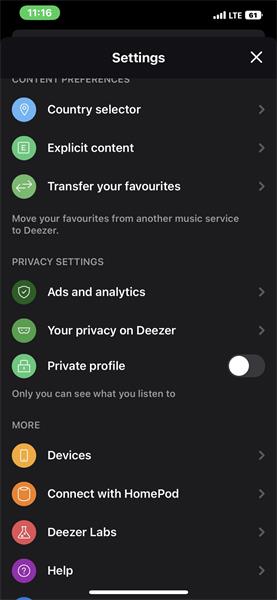**Detailed Caption:**

This image is a vertically-oriented screenshot resembling an Android or iPhone screen, set against a pitch-black background. On the top of the screen, there is a pitch-black status bar. In the upper left corner, a green oval displays the time "11:16" in white letters. To the right, there are four white icons: signal bars, an "LTE" label in all caps, and a battery icon showing the number "61" filled in with white.

Below the status bar, a dark gray bar contains the word "SETTINGS" in white letters, followed by a white "X" on the right. Descending further, "CONTENT PREFERENCES" is written in gray letters but gets partially cut off by the gray box below it.

Next, three circular icons are outlined. The first, a blue circle, contains a white location icon, accompanied by the words "COUNTRY SELECTOR" in white. To its right, a gray sideways-facing "V" indicates a submenu. 

Beneath it, a green circle features a white square with an "E" inside, with "EXPLICIT CONTENT" written in white to the right and another gray sideways "V". The next icon, a green circle with white arrows pointing left and right, is accompanied by "TRANSFER YOUR FAVOURITES" (using British spelling) to its right, followed by a gray "V". Below it, in white text, "MOVE YOUR FAVOURITES from another music service to DEEZER" is written.

Below this, "PRIVACY SETTINGS" is in gray, all caps. The following section shows a dark green circle with a white shield and checkmark, associated with "ADS AND ANALYTICS" to the right and a gray "V". A lighter green circle with white glasses follows, labeled "YOUR PRIVACY on DEEZER" also with a gray rightward-facing "V".

Next, a bright light green circle with a white padlock is labeled "PROFILE PICTURE" on the right. This has a unique gray oval with a white circle toggled towards "PROFILE" and "PRIVATE PROFILE," indicating it is toggled on. Beneath this, "ONLY YOU CAN SEE WHAT YOU LISTEN TO" is in gray text, followed by "MORE" in all caps.

Below "MORE," an orange circle with a white smartphone icon contains the word "DEVICES" to the right, with a rightward-facing "V". Further down, a slightly darker orange circle with a white cylinder icon labeled "CONNECT WITH HOME POD" has a gray "V" to its right. The next circle, light red with a white beaker, is labeled "DEEZER LABS" with a gray "V". Lastly, a purple circle at the bottom contains a white question mark with the word "HELP" to the right and a gray "V".

At the very bottom, a long, thick white bar spans the center. In the lower left, a partially cut-off blue circle is visible.